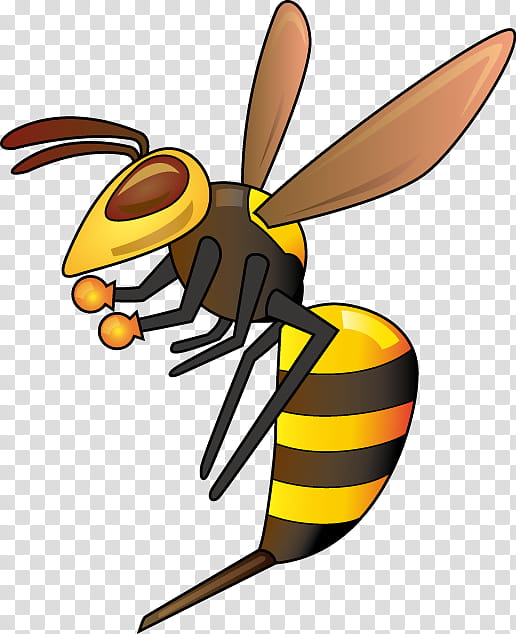This portrait-mode clip art image depicts a cartoonish bumblebee against a dark gray and white checkerboard background. The bumblebee, facing left, features a yellow head with a large, brown eye. Two dark red antennae, outlined in black, curve upwards from its head. Its body is adorned with alternating yellow and brown stripes leading to a plump abdomen. The bee has three pairs of black legs, with the front two pairs resembling little yellow boxing gloves. One wing is visible in the top right corner, light brown in color and outlined in black. This image, clearly designed for graphic applications, showcases the bumblebee's distinct markings and vibrant colors, making it suitable for use as clip art in documents or presentations about insects.